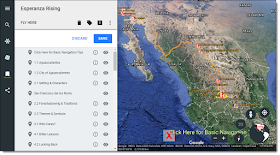The image features a horizontally oriented rectangular map, realistic in appearance, situated to the right of the frame. The map displays various geographical elements in detail, with a yellow path highlighting a specific route. The water bodies on the map are depicted in a gradient of blue, lighter near the shorelines which transition to green, and then to dark brown mountains towards the bottom of the image.

On the left side of the image, there is a vertical black navigation bar extending the full height of the frame. This navigation bar includes several icons, starting with a magnifying lens icon, followed by a star-shaped icon divided into four squares. Below these, there might be a home icon, indicated by a blue underline. Further down is a share icon, though the exact label next to it is unclear. Below these, there are additional icons, including one resembling a price tag and another blue button labeled "Save" in white text. There appears to be a list of items consistent with directions or steps, complementing the path visible on the map.